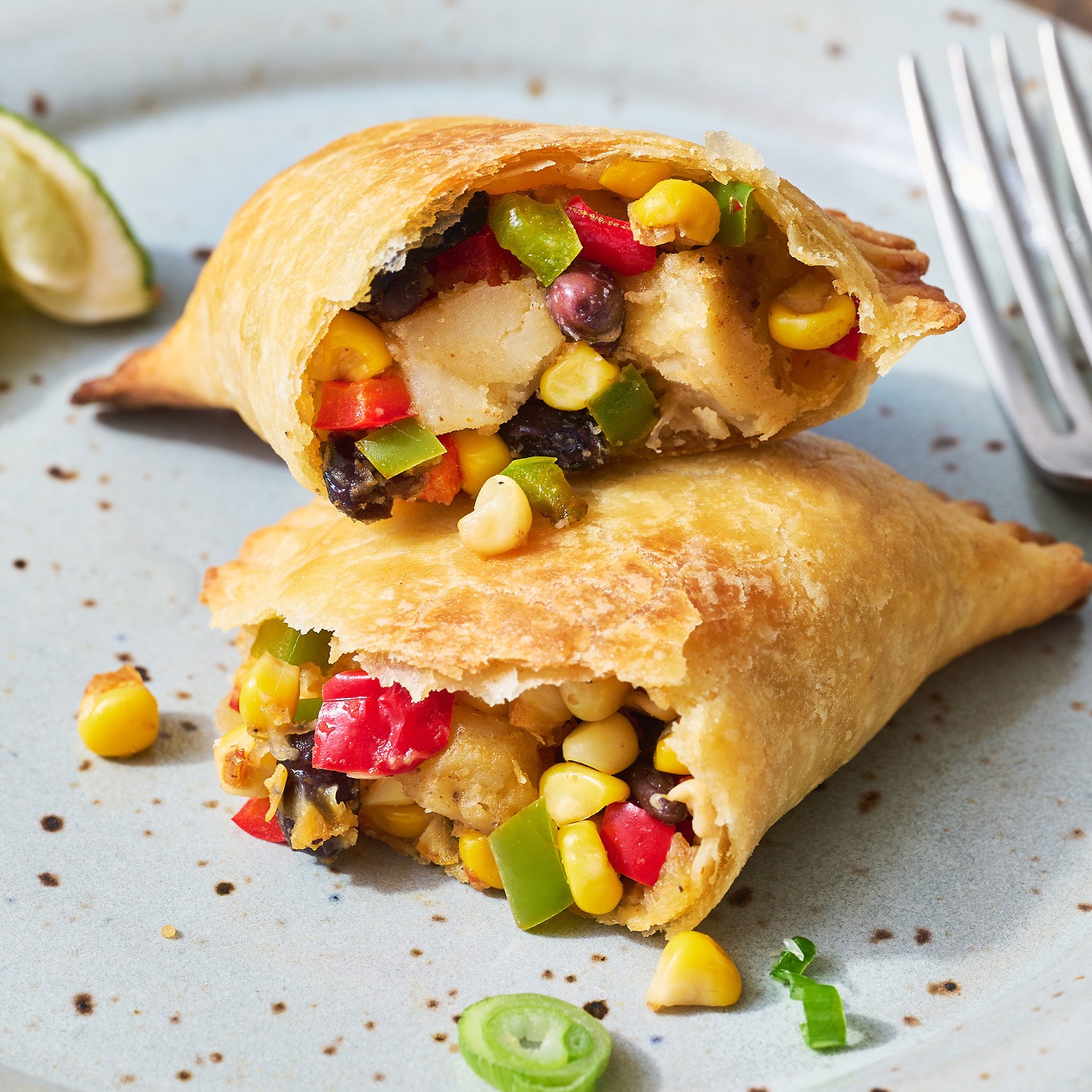This image features a close-up view of a torn-in-half pastry, possibly an empanada or pasty, with a flaky, yellowish-whitish crust. The inside reveals a colorful, mixed filling of various fruits and vegetables including yellow corn, green and red peppers, onions, black beans, and possibly potatoes, blueberries, and raisins. The bottom half rests on a speckled light gray plate, displaying its center filled with the aforementioned ingredients scattered about. The top half, also torn, is placed above, further exposing the vivid filling. To the top left of the image, a piece of a cut lime or avocado adds a splash of green, while the tines of a silver fork peek in from the upper right corner.